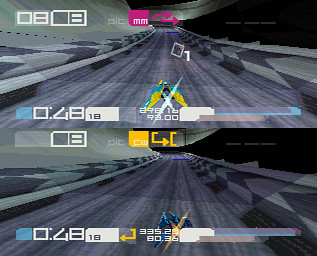This image showcases a split-screen view of a futuristic racing game. The screen is divided into two rectangular sections, one on top of the other, each displaying a different player's perspective. Both sections feature a sleek, concrete road with a modern, high-tech aesthetic. On the left side of each section, there are boxes displaying the time. The top section portrays a yellow and teal vehicle racing along the road, while the bottom section shows a blue and teal vehicle in action. The vivid colors and dynamic design elements suggest an exhilarating competition between the two players.